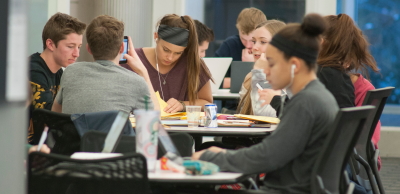The photograph features a bustling cafe or study area filled with predominantly well-dressed young people, who appear to be either college students or young professionals. At the forefront, a young African American woman with earphones sits at a white-topped table, focused on her laptop. A drink and some food are positioned nearby. To her left, a table hosts six students engaged in various activities—two men and three women, with one woman writing and others engrossed in their phones or conversing. The individuals around this table have a mix of materials and drinks spread out. In the background, two young men are visible, both with laptops open, contributing to the studious and collaborative atmosphere that pervades the scene. The entire space is furnished with black office chairs, adding to the organized and modern ambiance.